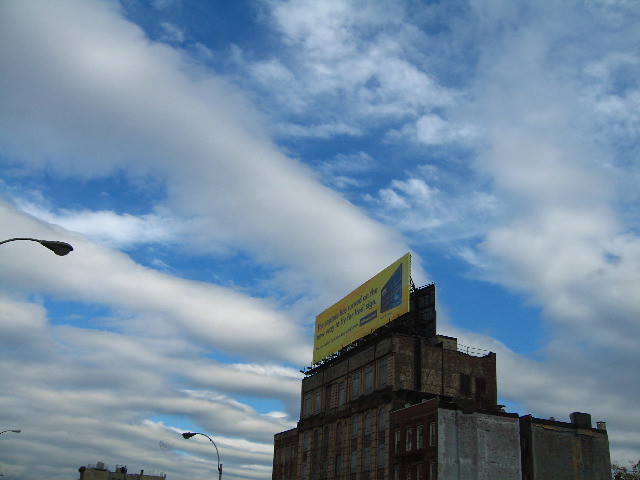A high-quality daytime photograph captures a vibrant urban scene. The sky is a stunning blue, adorned with thick, fluffy white clouds. A black streetlight stands prominently in the composition, juxtaposed against a large, architecturally diverse building. The building features a harmonious mix of brown, tan, and gray stone hues. Atop the structure is a striking billboard with a vivid yellow background, prominently displaying a blue credit or debit card on one side. Darker-colored text adds to the advertisement, while the supporting metal scaffolding is clearly visible. The building's windows vary in design, with some showcasing a rounded appearance and others adopting a more squared-off look.